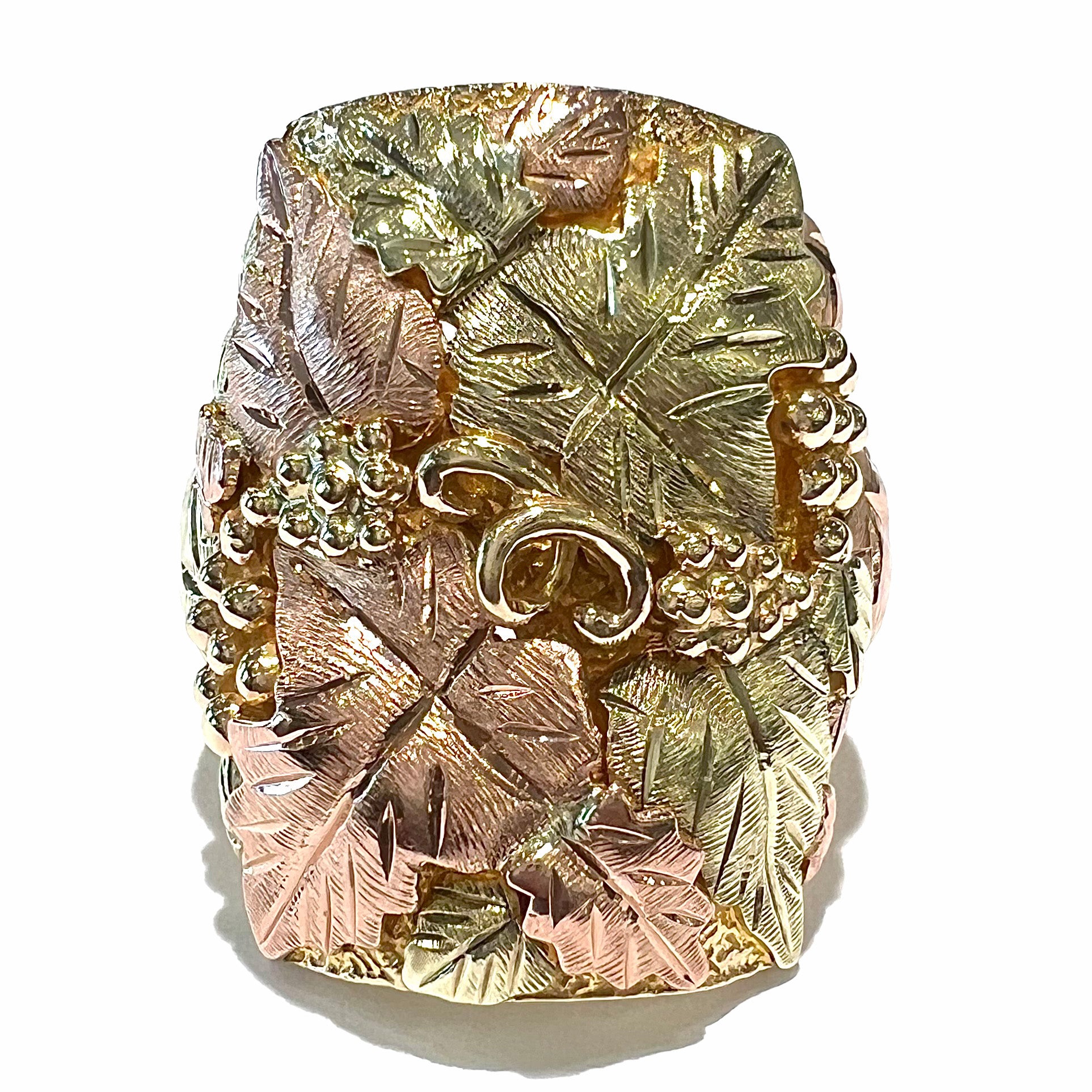This professionally-taken close-up photograph captures an intriguing piece of jewelry, likely a brooch, placed on a pure white surface with strong lighting that casts a distinct shadow behind it. The extravagant design is slightly taller than it is wide and features a slightly wider middle, displaying intricate and textured leaf motifs. These leaves come in various hues—including gold, coppery-pink, and greenish tones—each with lines etched on them that slant upwards. Scattered among the leaves are clusters of small, golden ball-like ornaments reminiscent of grapes. Dominating the center of the piece is a striking gold-colored coil, adding a swirl of elegance to the design. The overall impression is one of a vintage or antique item, boasting an elaborate, sparkly, and metallic appearance.